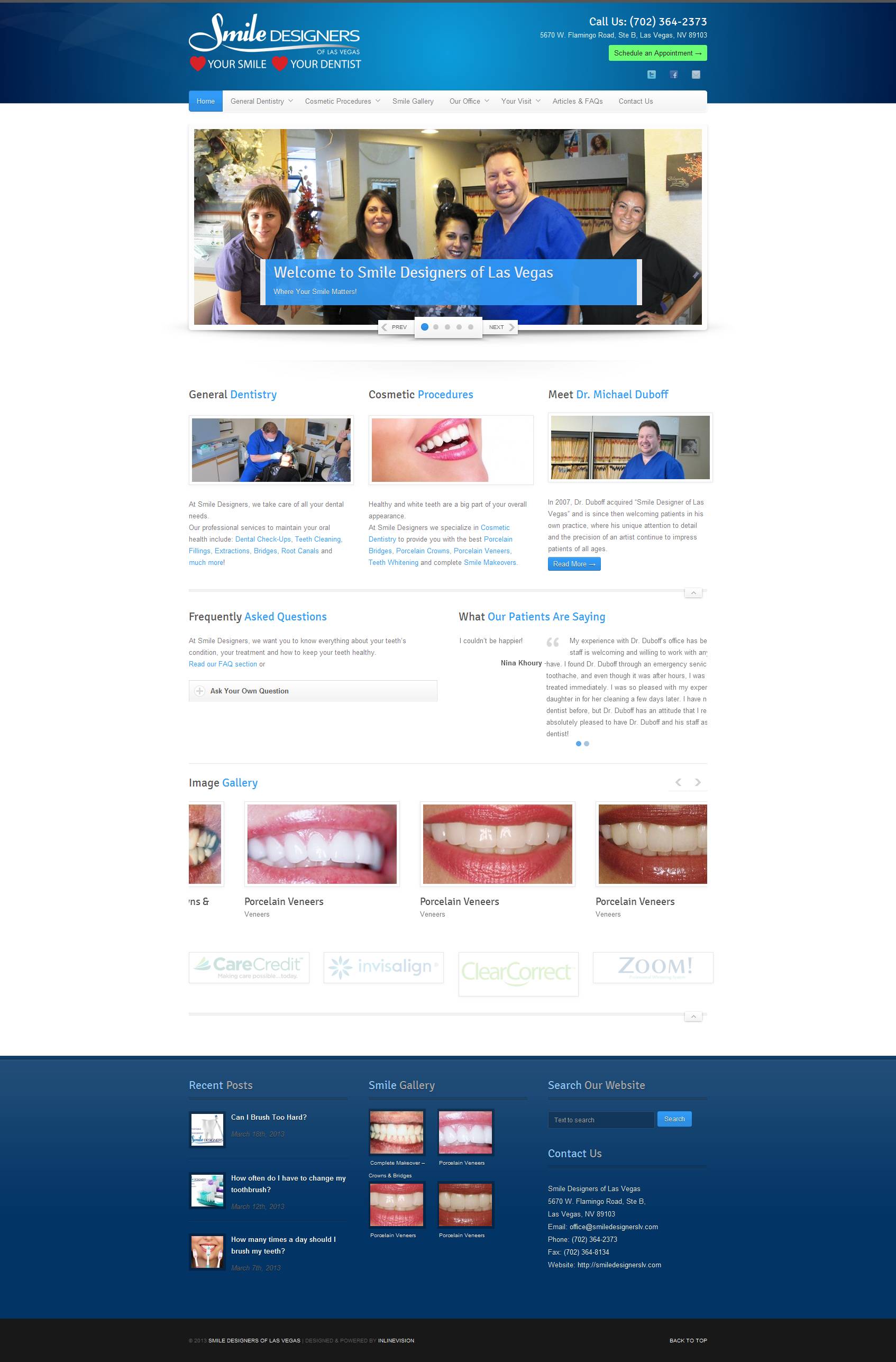**Detailed Caption for Website Image:**

The website for Smile Designers, a dentistry practice, prominently features the slogan "Your Smile, Your Dentist" adorned with two small heart icons beside each phrase. At the top right corner of the site, a blue banner displays the practice's street address alongside a telephone number, and includes a "Schedule an Appointment" button for convenience.

Below the banner, a welcoming photograph showcases the friendly office staff, consisting of four women and one man, all dressed in professional medical attire. They are smiling warmly in front of a backdrop of file cabinets, suggesting that they are situated in the front desk or administrative area of the practice where patients first check-in.

Scrolling further down the page, visitors can find sections detailing the range of services offered: general dentistry and cosmetic procedures. There is also a dedicated section to "Meet Dr. Michael Duboff," complete with the dentist’s name spelled out clearly (D-U-B-O-F-F).

An image gallery further down highlights the results of various dental procedures performed by the practice. The gallery features before-and-after photos of patients who have received treatments such as veneers. The images display a variety of outcomes, ranging from super white veneers to more natural-looking shades, showcasing the versatility and personalized care offered by Smile Designers.